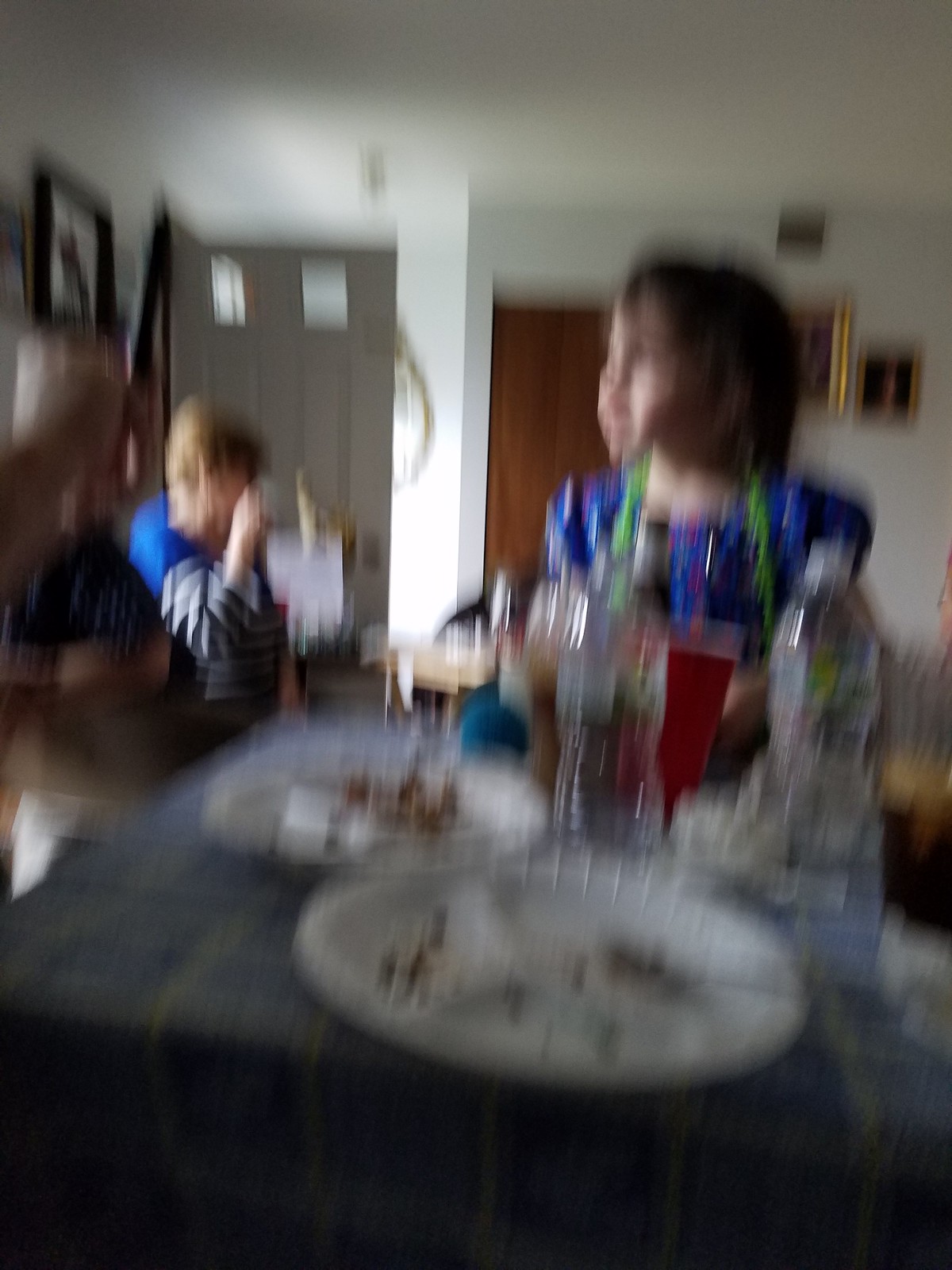A blurry photograph captures a bustling indoor scene of people enjoying a meal together. The setting appears to be a cozy living room, adorned with gold-framed pictures on the walls and a wooden closet door in the background. Light filters in gently from the front door, adding a warm ambiance to the room. Central to the image is a table covered with a navy tablecloth, scattered with styrofoam plates, clear plastic water bottles, and red Solo cups, suggesting a casual and relaxed gathering. Among the diners, a person in a blue shirt with white and black stripes is seated off to the side, while a child is visibly enjoying the meal at the table. Though the motion blur adds a sense of lively movement, the essence of a convivial gathering remains evident.